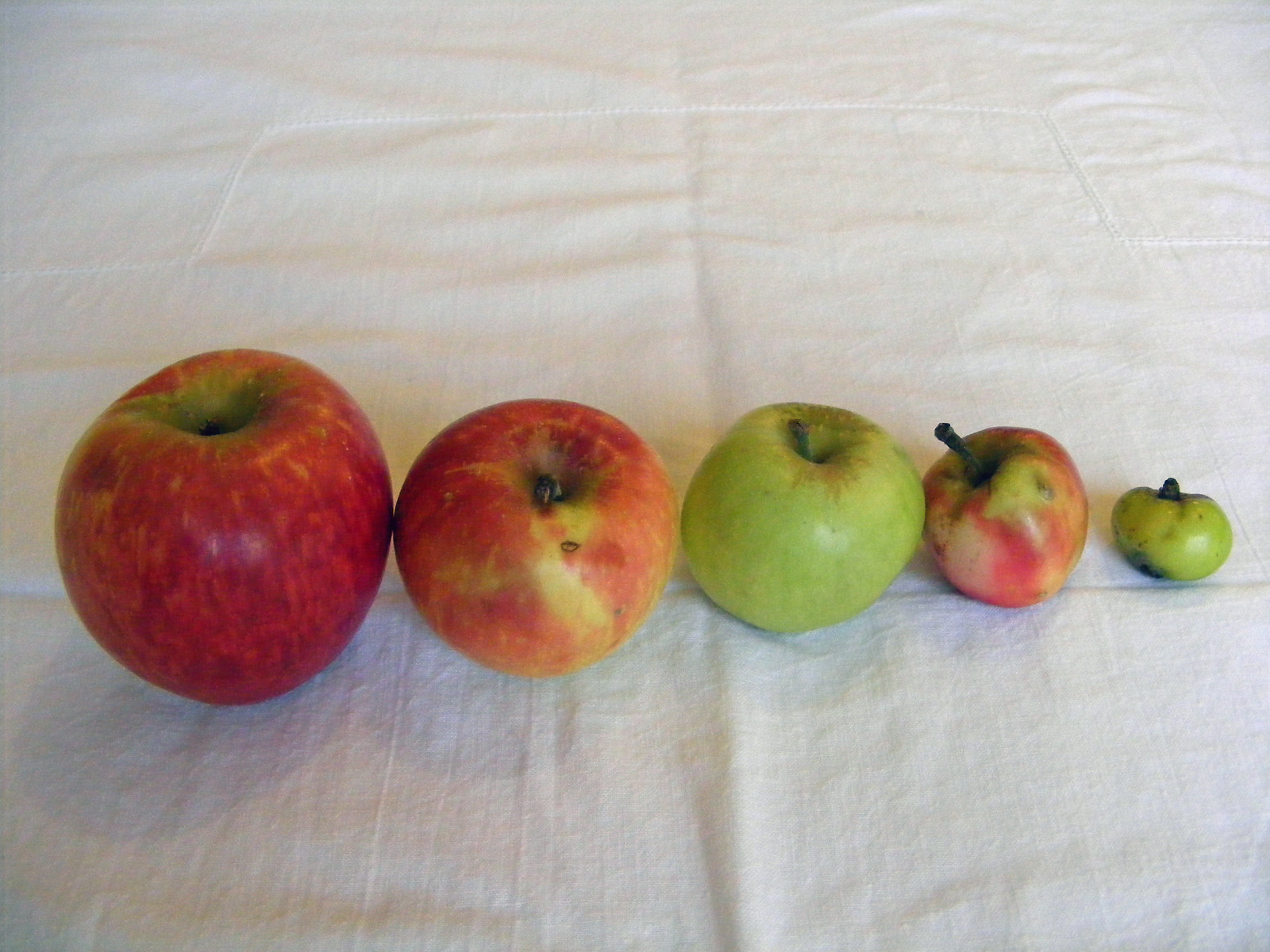The image showcases five apples arranged horizontally on a white cloth bearing a floral pattern, resembling a tea towel. Starting from the left and moving right, the apples decrease in size. The first apple on the left is the largest, predominantly red with a touch of green near the stem. Next to it is a slightly smaller apple that is yellowish-red. Following this is a medium-sized green apple. The fourth apple is another red one with more noticeable green areas, slightly smaller than the previous apples. The fifth and final apple on the far right is the smallest, very green, and carries a faint hint of black. The apples' gradient sizes and varying colors create a balanced, aesthetically pleasing composition against the intricate floral backdrop.